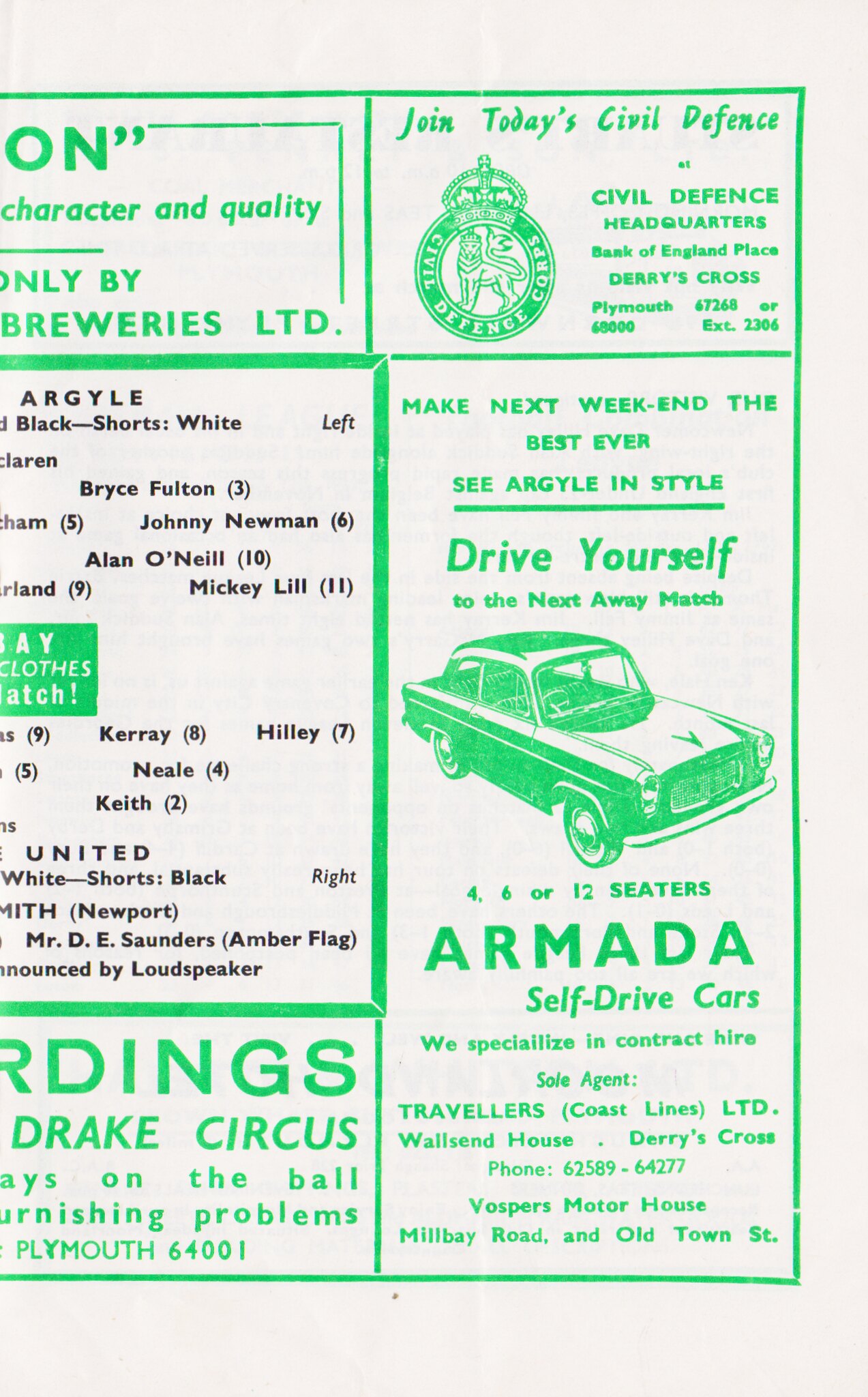This image appears to be a scan of a page from an old British football program, likely focusing on advertisements. The page is white with primarily green printed content, except for one section with black text. The layout is divided into six distinct sections.

In the top right, there's an advertisement urging readers to "Join today's civil defense," providing details such as the civil defense headquarters at Bank of England Place, Derby's Cross, and featuring the Civil Defense Corps insignia, which includes a central lion motif. 

Directly below is an ad promoting Armada self-drive cars, encouraging fans to "Make next weekend the best ever" by driving themselves to the next away match in style. This section includes a drawing of a classic 1950s-style car and mentions their specialization in contract hire.

On the left column, there are three ads, though partially cut off, suggesting there could be a missing page. The top one highlights "Character and Quality." The middle ad is likely a roster for the team, containing detailed information about players under the heading ‘Argyle.’ The bottom ad talks about "Drake Circus," possibly related to a brewery or local business.

Overall, the page offers a nostalgic glimpse into the era of classic advertisements intertwined with local football culture.